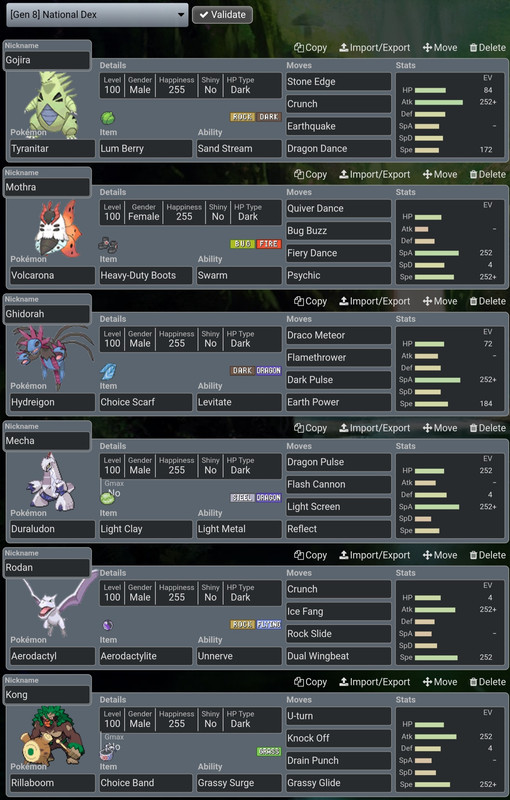This screenshot captures a portion of the Pokédex from a Pokémon game, specifically categorized as Gen 8 within the National Dex. A "Validate" button with a white checkmark is positioned adjacent to these labels. At the top of the list, the Pokémon named "Gojira" stands out. It is a Level 100 male with maximum happiness of 255 and is identified as shiny. Additionally, it has no hidden power type and is classified as dark. Below Gojira, another Pokémon named "Mothra," recognized as Volcarona, is displayed. Each Pokémon entry is accompanied by detailed stats and characteristics on the right-hand side of the screen.